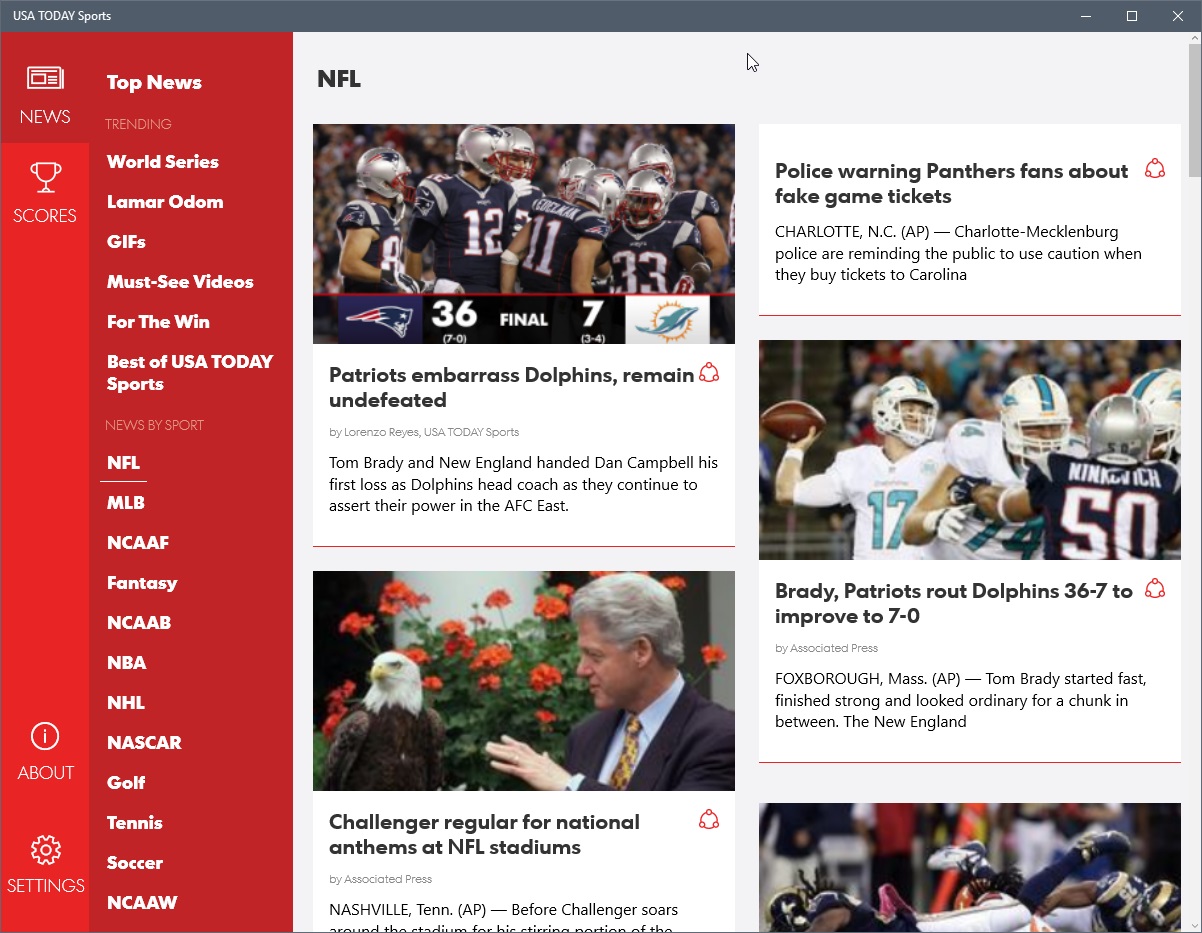This image captures a cropped screenshot of the USA Today Sports section on their desktop website interface. On the left side of the webpage, a prominent vertical red panel features distinct sections and icons, each demarcating different navigation categories. At the top of this red panel, "Top News" is prominently displayed in bold white letters, with "Trending" appearing below it in much smaller white text. This panel continues down the page, listing various categories. 

In the top left of the red panel, there's an icon resembling a newspaper with the label "News" underneath. Directly below, an icon of a trophy accompanied by the word "Scores" in smaller white letters appears. Near the bottom left, an eye icon is shown with "About" positioned beneath it, and at the very bottom, a cogwheel icon is labeled "Settings."

To the right of this vibrant red navigation panel, the main body of the webpage features a gray background. At the top left of this section, "NFL" is prominently displayed in bold black letters. Below this heading, various articles are presented, each accompanied by photo thumbnails, creating a comprehensive and visually organized overview of the latest sports news.